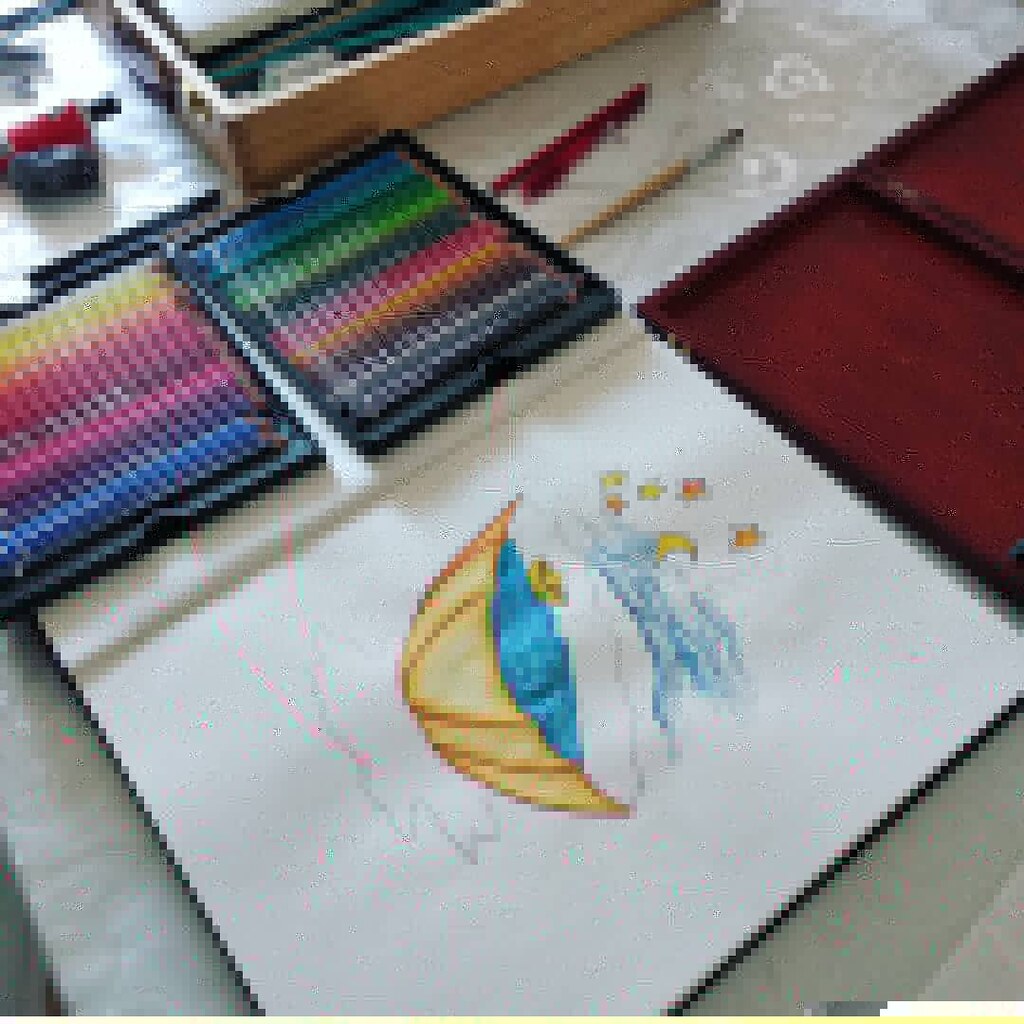A blurred photograph showing a white drawing tablet trimmed in black positioned on a surface, possibly a white tablecloth with a shiny design. On the tablet, there's an indistinct drawing that resembles an umbrella with a yellow half-round shape bordered in a darker yellow, filled in with blue, and accented by blue, white, and gray elements. Several small dots of yellow, red, and orange scatter across it. Surrounding the tablet are various objects: on the upper left, there’s a beige wooden box with green and white contents, which might include green pencils. To the right of the tablet, there are cases filled with colored pencils of multiple hues—blue, green, light green, purple, light purple, pink, yellow, black, gray—and variety of red, blue, and yellow pencils scattered about. Additionally, a red pen lies outside two black cases of pencils. Above these items is an indistinct red object, possibly a burgundy red box, and at the bottom center, there's a red and grey object with something black adjacent to it. Everything in the scene appears quite blurred, making the precise identification of some items challenging.